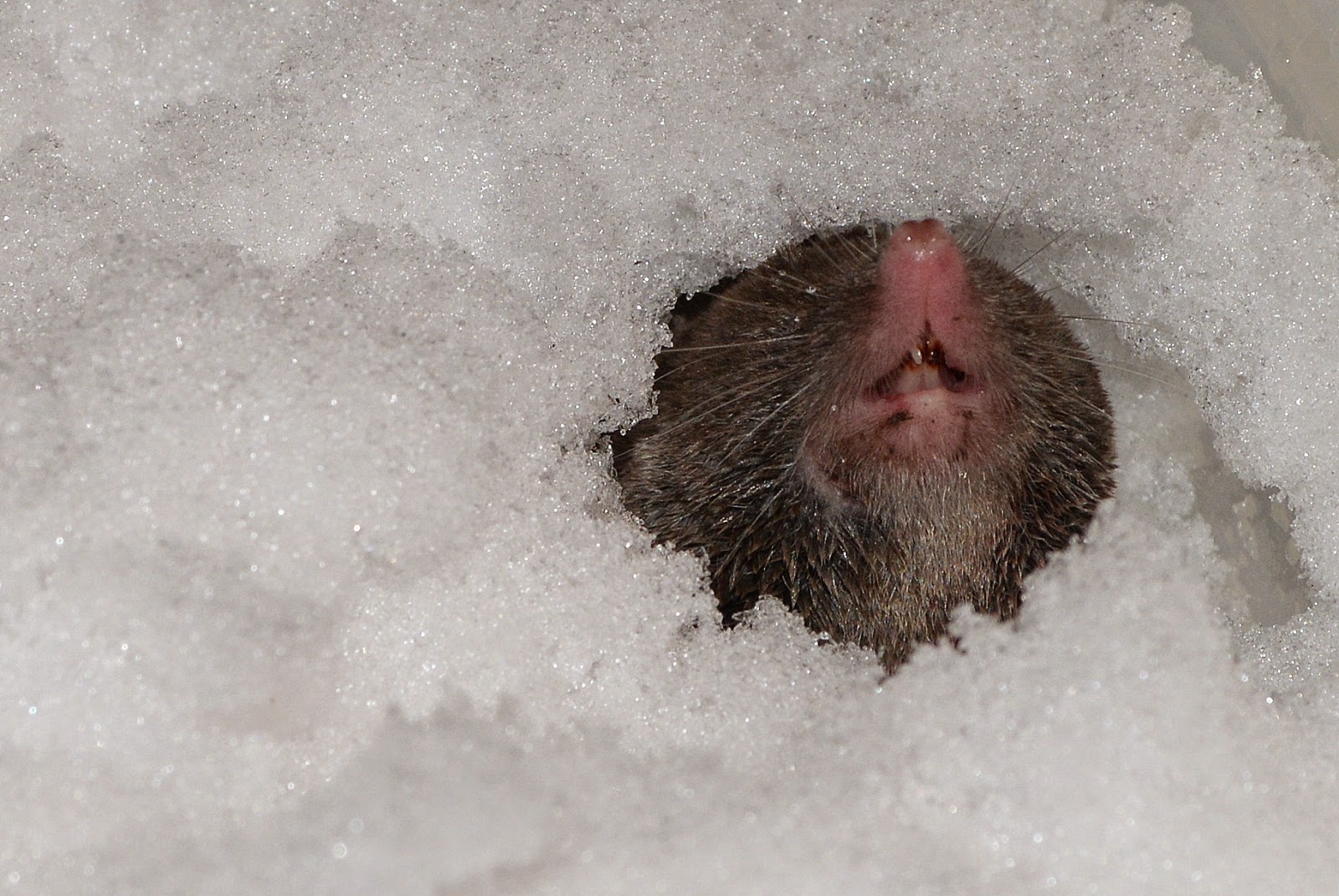The image depicts an animal cell beneath a layer of what appear to be melting snow or ice crystals. The scene is dominated by bright white, shiny crystals scattered around, interspersed with tiny gray shadows that enhance the overall whiteness and sparkle of the setting. Towards the right side, a small hole reveals a pink snout with two visible teeth, surrounded by a circle of brown fur and delicate whiskers. The creature's eyes are not visible; only the underside of its mouth and nose can be seen. The face, with its fur and distinctive features, peeks out from the surrounding icy crystals, creating the impression of an animal, possibly a raccoon, partially buried in snow. The red coloring of the snout and mouth area contrasts with the white expanse, adding detail to the buried face, while the overall environment gives a cold, wintry feel to the shot.